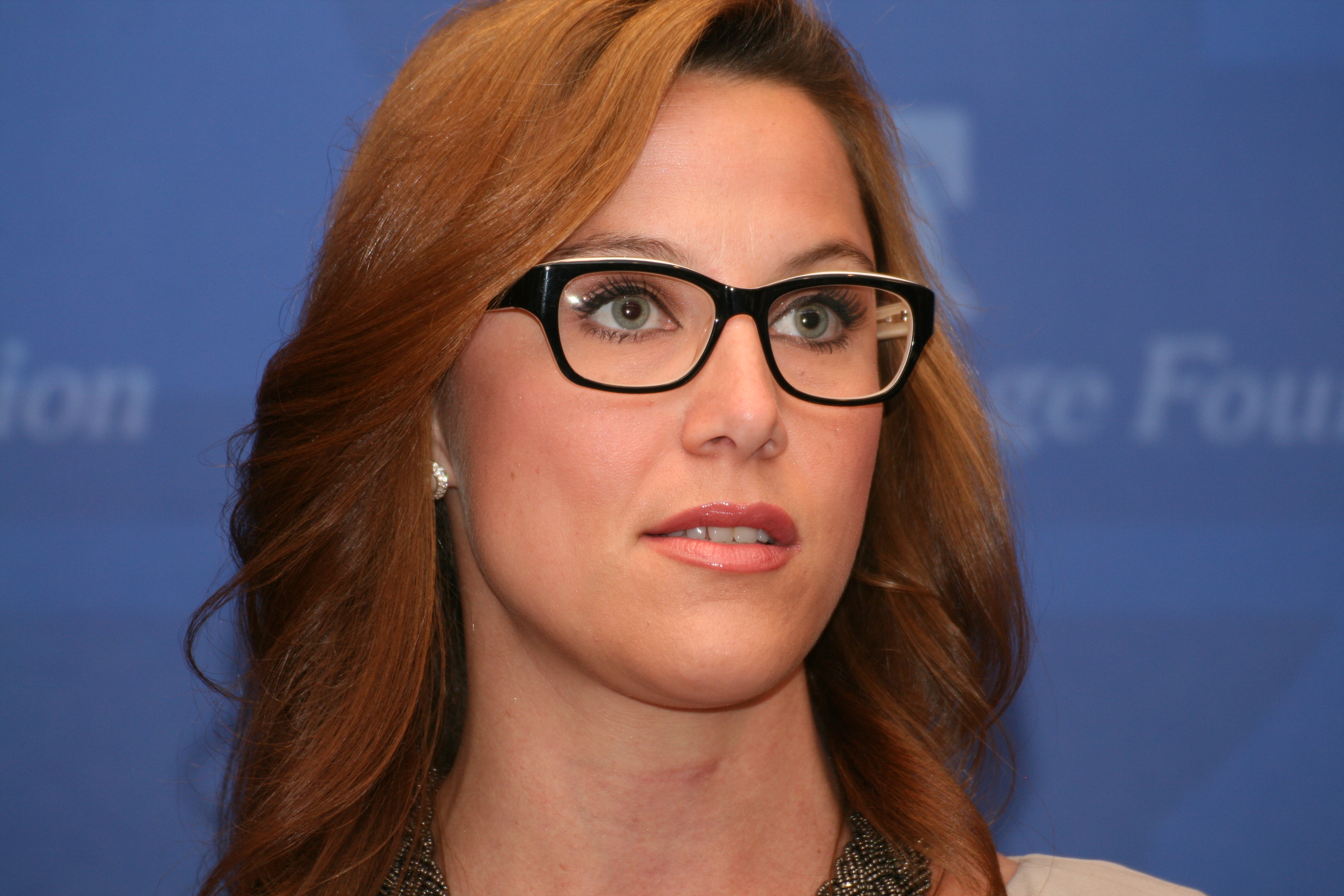The photograph captures a woman in her 30s or 40s standing against a blue backdrop adorned with partially visible white letters that read "ON" on one side and "G-E-F-O-U" on the other. The woman has slightly curly, shoulder-length brown hair, possibly dyed, which some might perceive as a muted red or ginger hue. She is donned in a tan-colored top paired with a thick, interwoven metallic necklace, and is accessorized with round pearl earrings. Her black, plastic-rimmed glasses with clear lenses frame her pale green or hazel eyes, which look off to the right as if she is intently listening or involved in a conversation, captured in a candid moment. Her minimal makeup emphasizes her natural features, and her expression is neutral with her slightly open mouth showing a hint of teeth.